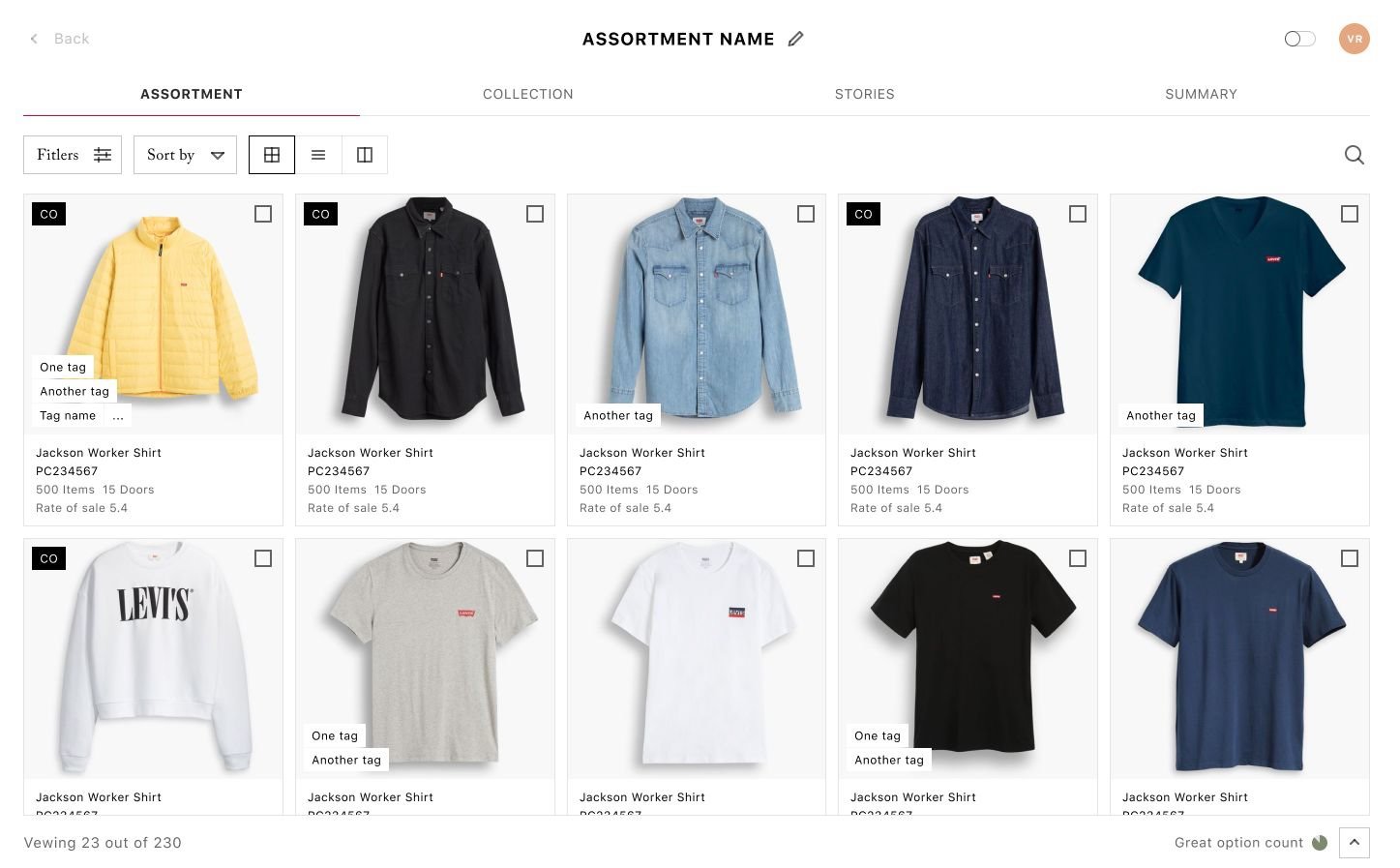Here is a detailed and cleaned-up caption for the image:

---

The screenshot captures a retail website focused on selling tops, prominently featuring the site name "Assortment Name" at the top center, accompanied by a pen graphic on the right. The page displays four tabs at the top, with the currently active tab being "Assortment," highlighted by a purple underline on the left side. Directly below the assortment tab, several elements are visible: a filters box, an "Assort by" box, and three additional icons likely related to page layout options.

The main content area is organized into two rows of various shirts, showcasing both long sleeve and short sleeve options. The first item, a "Jackson Worker Shirt," appears as a yellow jacket and is marked with a "CO" tag in the top left corner. This item has a rate of sale listed as 5.4. In the second row, the initial item is a "Levi's Worker Shirt," also featuring a "CO" tag in the top left corner. Below these rows, text indicates that the viewer is seeing 23 out of a total of 230 items. In the far right corner of the page, there is an off-toggle slider and a profile avatar labeled with "VR."

---

This revised caption provides a clear, structured, and comprehensive description of the screenshot.